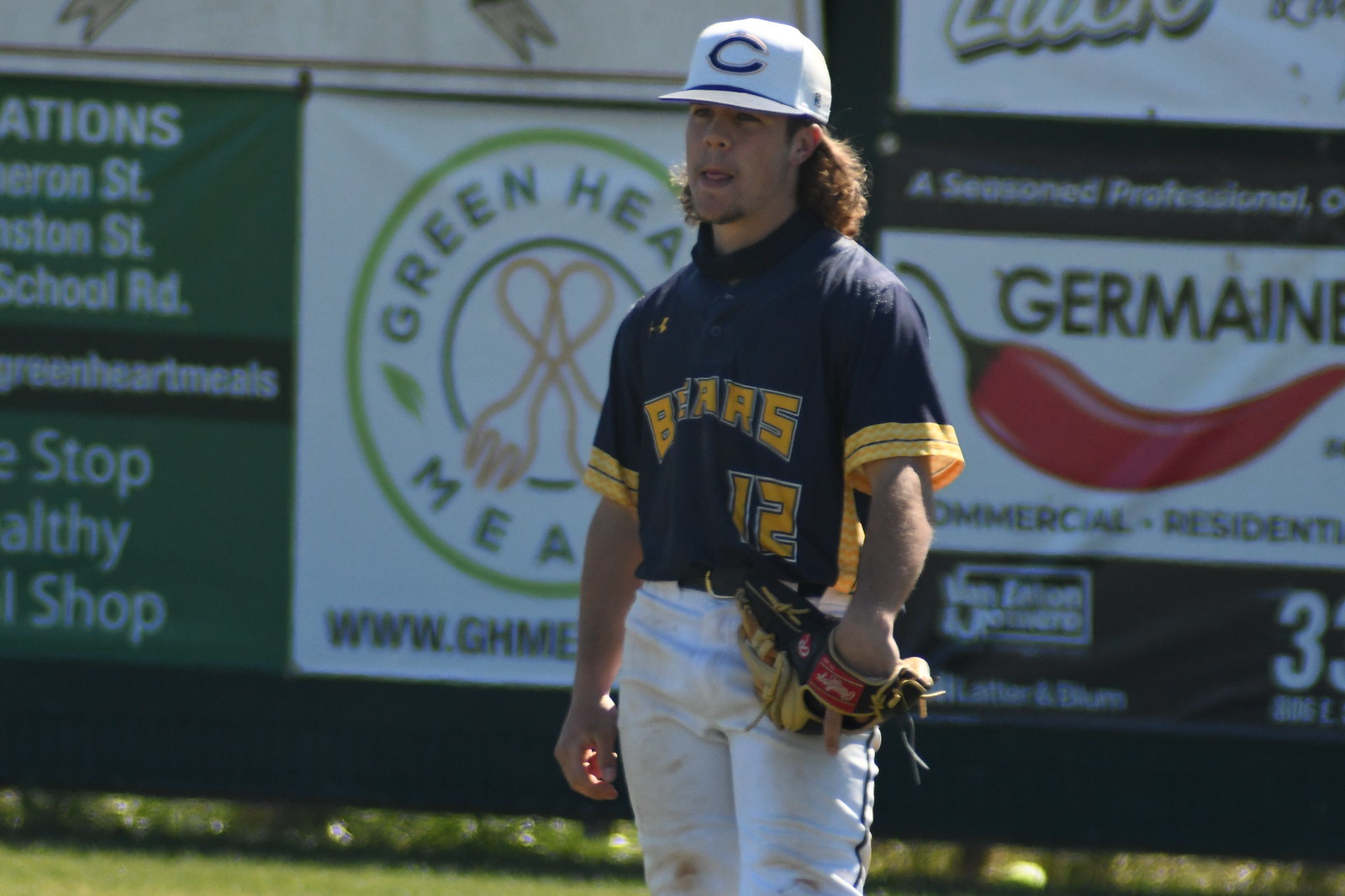This detailed, close-up color photograph captures a baseball player standing in the outfield. He is clad in white baseball pants with blue pinstripes down the sides, which are smudged with brown dirt, suggesting he has been sliding or diving. The player sports a blue and yellow striped jersey with "Bears" emblazoned in yellow across the chest, and the number 12 beneath it. Topping off his uniform, he wears a white hat featuring a prominent blue "C." With his Rawlings glove resting on his hip, his long brown hair peeks out beneath his cap. The backdrop of the image includes a large green wall adorned with multiple sponsor advertisements, among which a large red chili pepper labeled "Jermaine" and images of forks and spoons are distinguishable.